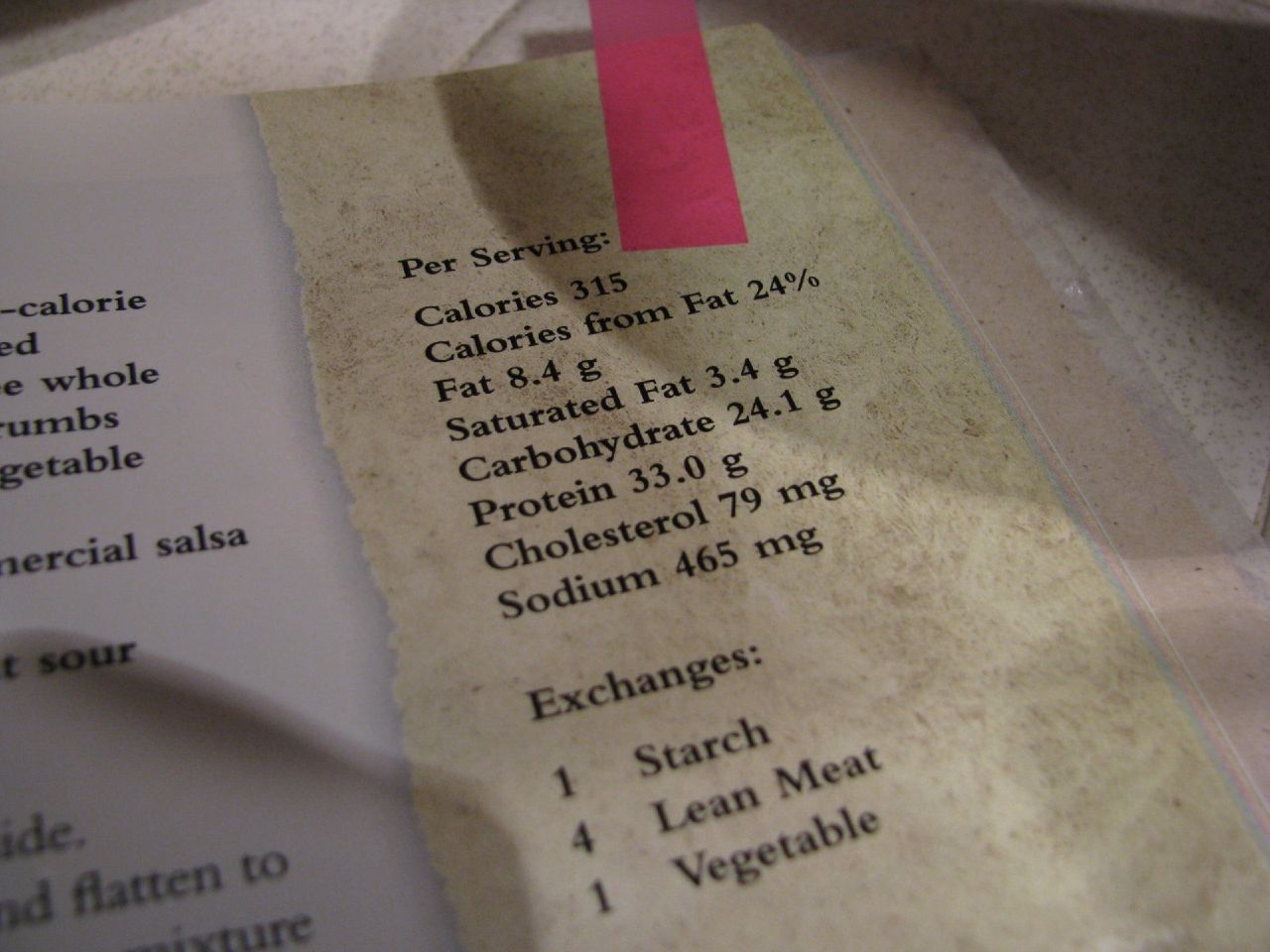The image is a close-up of a page from a recipe book, specifically highlighting the nutritional information per serving. The prominent nutritional facts include 315 calories, with 24% from fat, 8.4 grams of fat, 24.1 grams of carbohydrates, 33 grams of protein, 79 milligrams of cholesterol, and 465 milligrams of sodium. Additionally, it indicates exchanges corresponding to one starch, four lean meats, and one vegetable. The page seems weathered and has been placed on a white, hard surface with black specks. The text is positioned on the right-hand side of the page, with a partially visible recipe on the left showing fragments like "salsa," "sour," "whole," "crumbs," and "vegetable." Notably, the top features a pink sticky note tab for easy identification.